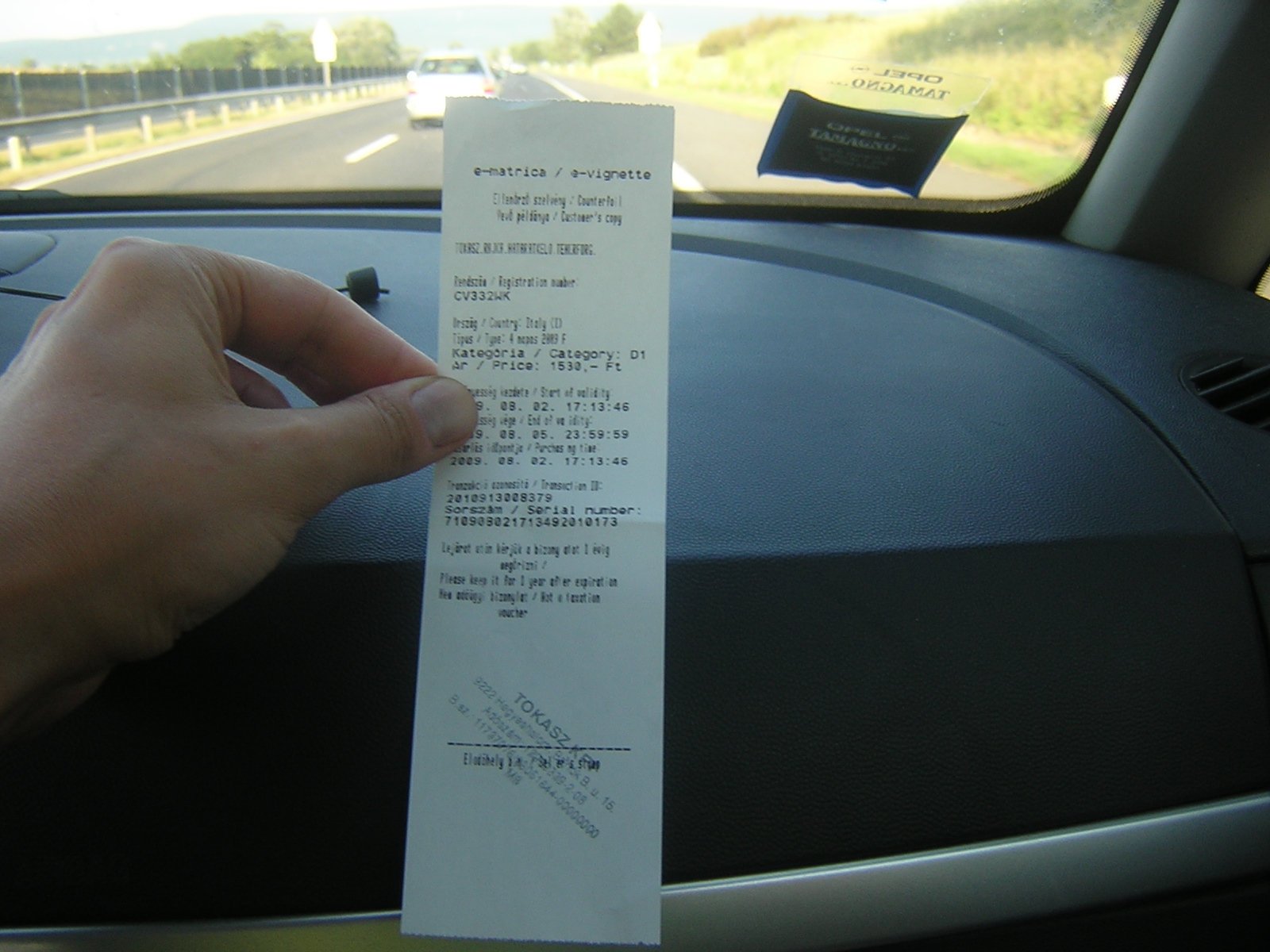The image captures the interior of a car, with the focus on a person seated in the passenger seat holding up a white receipt. The receipt, although somewhat difficult to decipher, appears to be from an establishment possibly named "E. Matricia" or "E. Vignette," and it lists several purchased items, likely in a foreign language. The bottom of the receipt features a signature line with an illegible inscription beginning with "TOKASZK," accompanied by what seems to be a company stamp.

The car's interior presents a two-tone design, with a black upper section and a silver or gray lower section. Ahead of the car, a white vehicle travels on a two-lane highway. To the right of the scene, expansive grassy hills stretch out, while large, dense trees loom in the distance, framing the road and adding a scenic touch to the otherwise mundane setting.